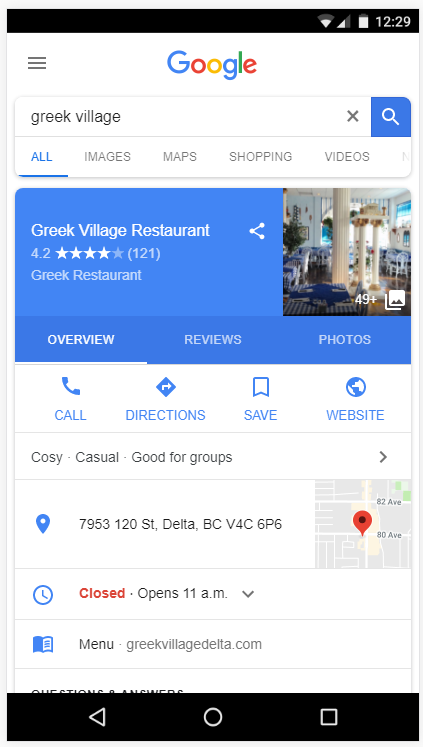The image is a screen capture from a mobile device displaying a Google search results page. The Google logo, featuring its signature blue, red, yellow, and green colors, is prominently positioned at the top. Below the logo, the search bar contains the text "Greek village." 

Directly under the search bar, the page offers quick access tabs: "All" highlighted in blue, and the options "Images," "Maps," "Shopping," and "Videos" in gray. 

The main content shows search results for "Greek village restaurant" displayed on a blue background with a corresponding image to the right. Beneath this, there are quick action buttons for "Call," "Directions," "Save," and "Website," all in blue.

Further down, there is a description: "Cozy, casual, food for groups," in black text. The listing also provides the restaurant's location and operating status, indicating "Closed" in red text. It notes that the restaurant "Opens 11 a.m." with a drop-down arrow adjacent to the opening time.